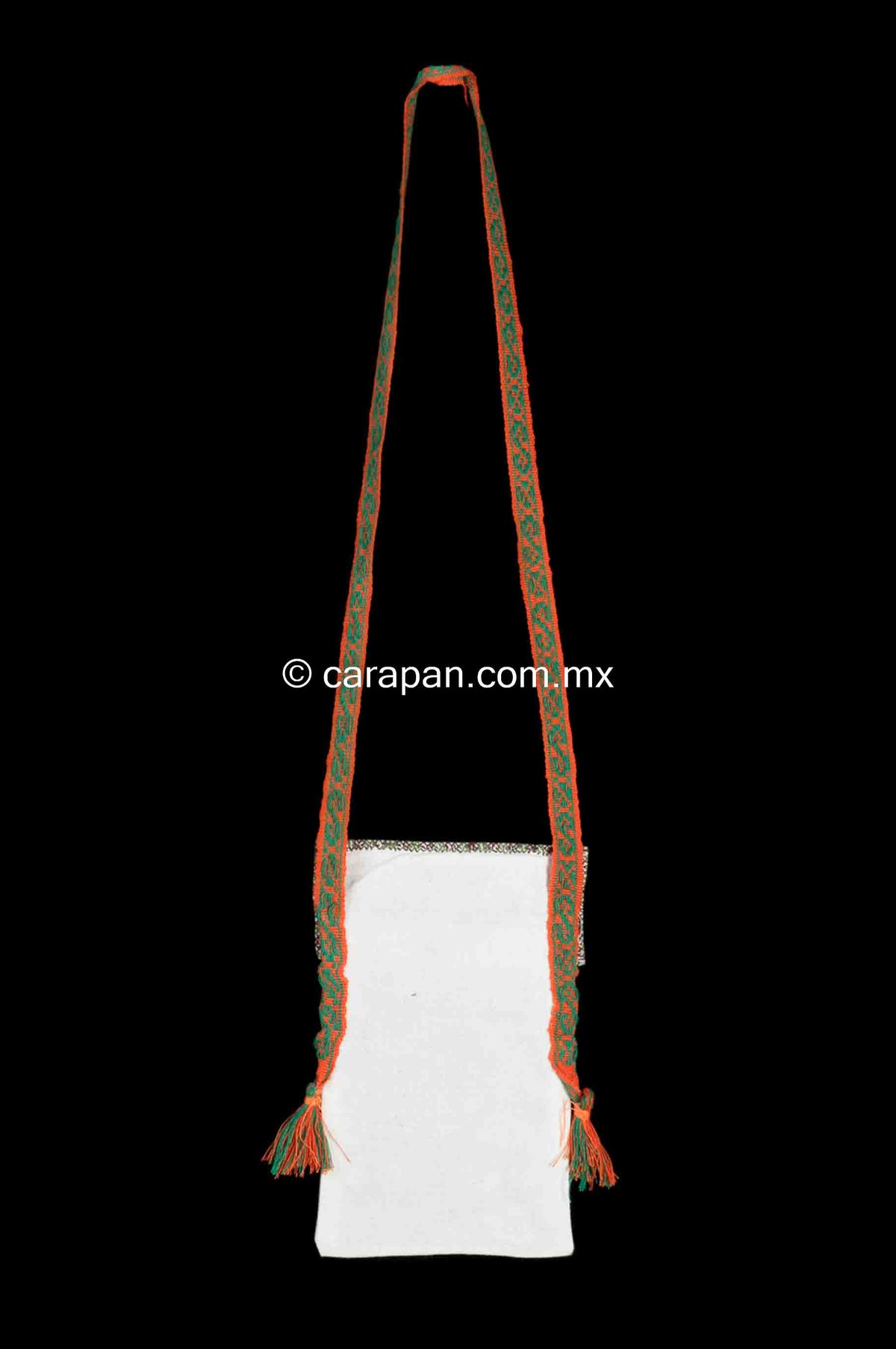This image displays a detailed product photo of a fabric item against a completely black background. The fabric item appears to be a tall, vertical rectangular-shaped white canvas bag, adorned with intricate embroidered designs in purple and green across the top. Attached to the bag is a long, decorative strap, predominantly orange with medium green inserts. The strap features an elaborate woven pattern composed of several repeating green 'S' shapes, creating a geometric look. The strap extends upwards from one side of the bag, loops at the top of the image, and descends back down to the other side, indicating that it is likely hanging from a point above. This strap also has tassels tied at its ends. The combination of colors, primarily red and green, may suggest a celebratory or academic significance, perhaps used with a graduation gown to denote a master's degree or PhD. Over the strap is a white text that reads "copyright carapan.com.mx," ensuring the item's copyright is stated explicitly. The overall intricate craftsmanship and design suggest a significance of ranking, royalty, or festive celebration.